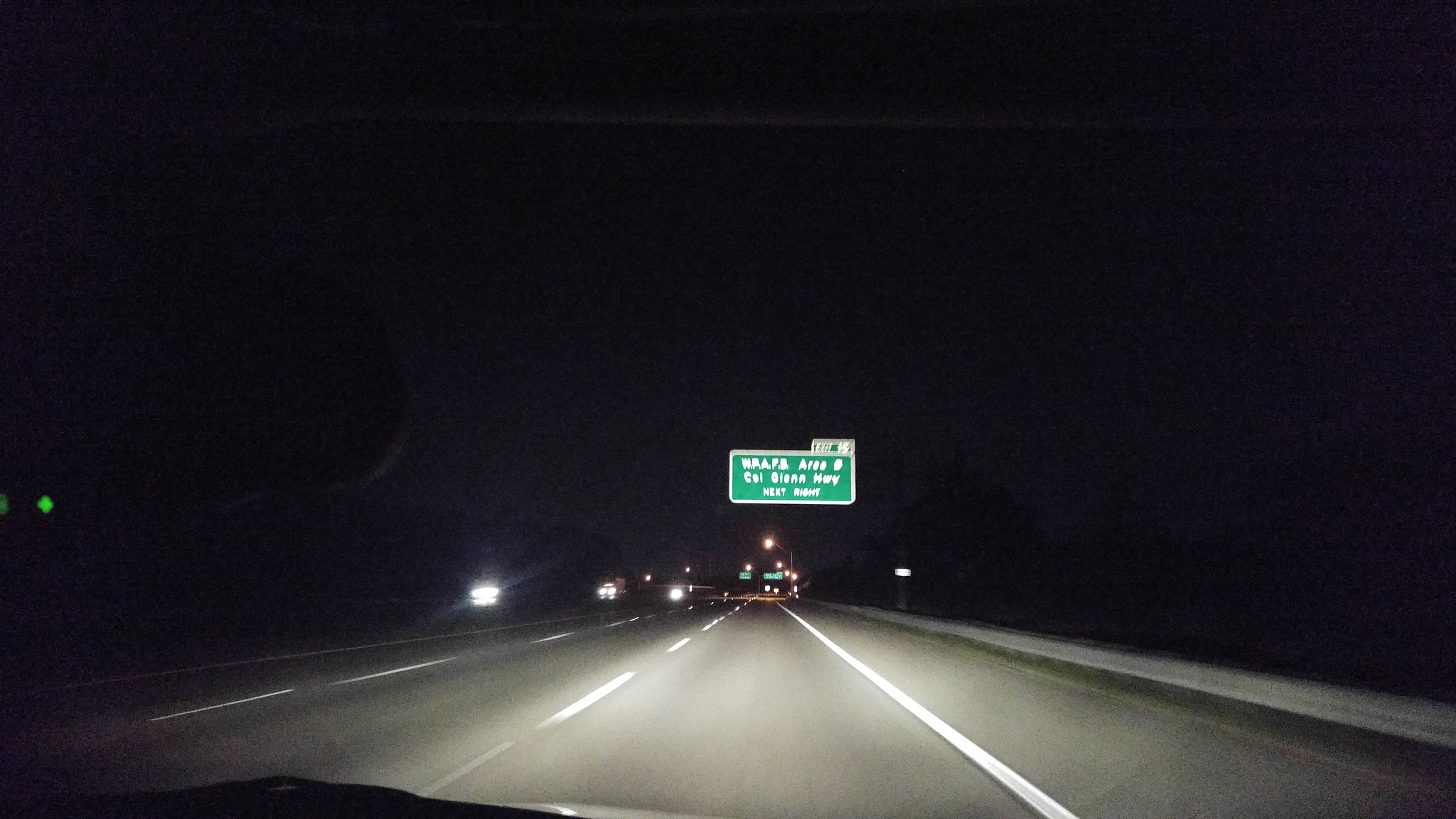This photograph, taken from inside a car on the passenger side, captures a nighttime view of a multi-lane highway. The bottom left corner of the image reveals a small portion of the car, including the rearview mirror and windshield wiper. The road ahead, illuminated by the car's headlights, features a silverish surface with both solid and dotted white lines marking the lanes. In the distance, a green, rectangular highway sign hovers overhead, adorned with blurry white letters likely indicating "COL Glen Highway, next right," although the top words are too unclear to decipher. The dark sky emphasizes the nighttime setting, with additional green diamond lights visible on the rearview mirror. Various lights from other vehicles, including headlights from cars approaching in the opposite direction on the left, add to the scene's authenticity, along with dark shadows of trees lining the road.